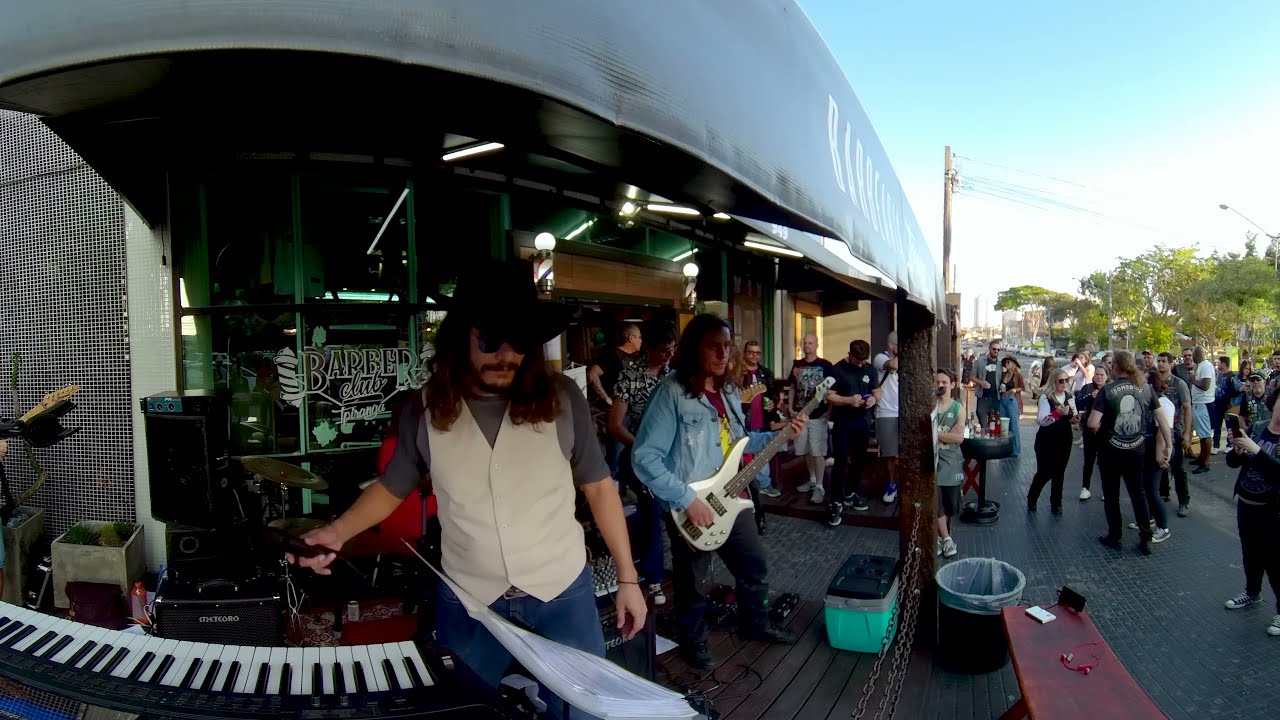This detailed photograph captures a vibrant outdoor scene set in front of a barbershop or club named "Barbers Club" or "Barber's Club Cafe." Viewed from a side perspective on the corner of the establishment, the setting features a musical performance under an overhang with a rock or country band as the focal point. The venue has a wraparound trim at the top, displaying the establishment's name in white paper letters on a black background.

At the center, band members are actively playing: one performer with long brown hair, black hat, shades, and a white vest over a gray shirt, is playing a white guitar, while another band member with equally long hair is donned in a blue jean shirt and blue jeans, playing the keyboard. Accompanying them in the background are speakers, a drum set, an ice chest, a trash can, and a red bench.

The scene is bustling with various individuals milling about. To the right, an audience listens to the music, with one lady capturing the performance on her camera, amidst numerous people casually walking and interacting in different directions, suggesting a festive or casual gathering. Cars are sporadically parked, and the right part of the image features sky views, electrical wires, and some trees, encapsulating the lively ambiance of an outdoor musical event.